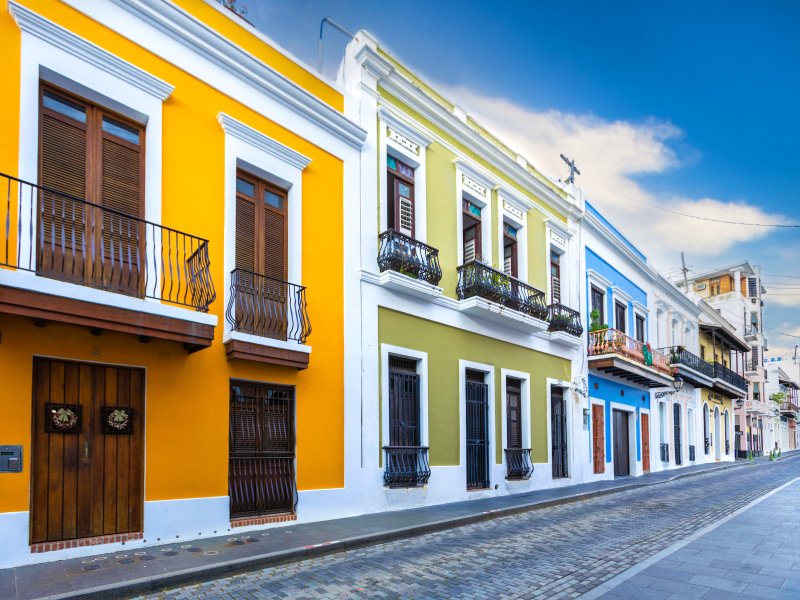A vibrant, full-color photograph captures a serene, well-kept city neighborhood street on a sunny day with clear blue skies and a few fluffy white clouds in the center. The street, made of cobblestones, stretches out from the bottom of the image and is devoid of traffic and people, enhancing the calm atmosphere. Lining the street are beautifully maintained two-story townhouses, showcasing a range of vivid colors including orange, lime, blue, white, tan, and others. The townhouses exhibit charming old Spanish architectural details with wrought-iron balconies, some adorned with plants, and heavy wooden French doors. The upper stories feature open windows and doors with wooden shutters, while some lower windows are protected by iron bars. This charming scene evokes the aesthetics of South American or Caribbean locales, reminiscent of places like Cartagena or old San Juan, despite their global architectural parallels.